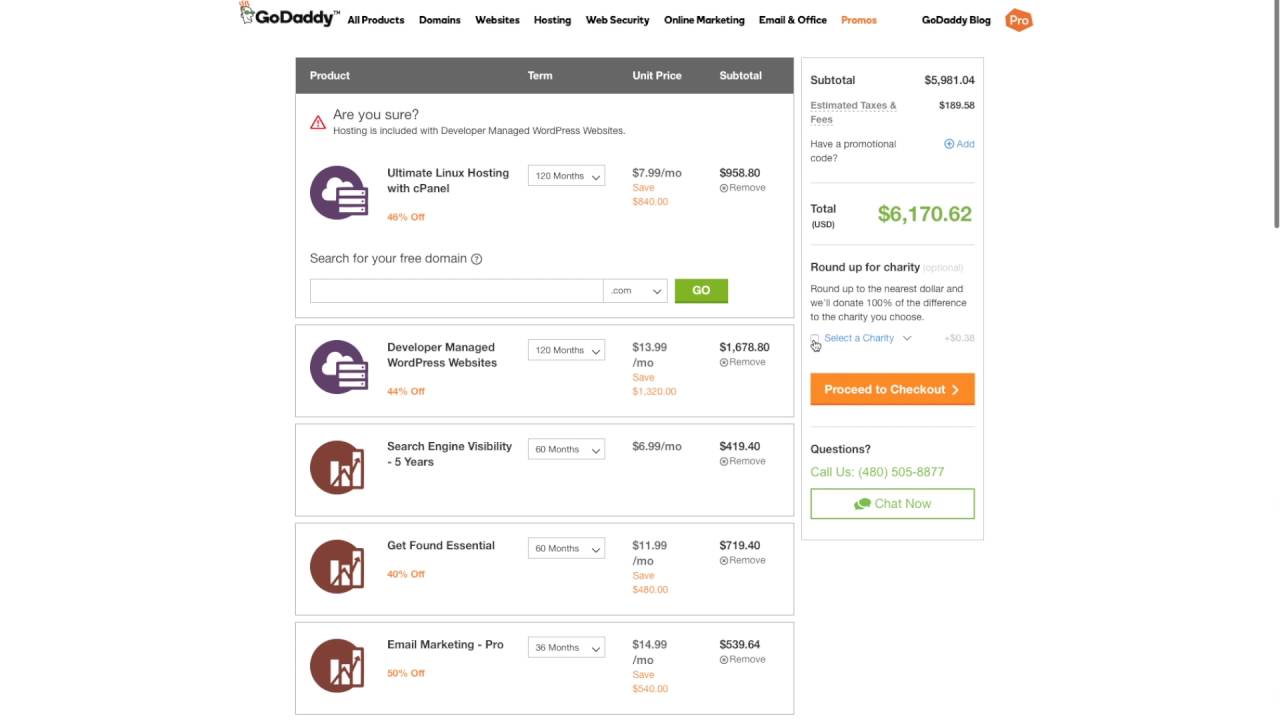This screenshot captures a GoDaddy website interface displayed on a desktop or laptop browser. The header, set against a white background, prominently features the GoDaddy logo on the top left, followed by a navigation menu. The menu includes links to various sections: 'All Products,' 'Domains,' 'Websites,' 'Hosting,' 'Web Security,' 'Online Marketing,' 'Email & Office,' and 'Promos' with the latter highlighted in orange. On the top right, the header displays 'GoDaddy Blog' in black text, accompanied by a small orange hexagonal icon with the word 'Pro' written in white.

The main content of the page is divided into two sections. On the left side, there is a list of various website-related products available for purchase. The right section features a vertical, rectangular invoice displaying a breakdown of the purchase. The invoice shows a subtotal of $5,981, with additional taxes and fees bringing the total to $6,170.62, prominently displayed in large green font. Beneath the total, there is a blurb about charity followed by a 'Proceed to Checkout' button in white text on an orange rectangle. Below this, there is a 'Questions' section with a green 'Chat Now' button and a phone number for further assistance.

The entire webpage is cleanly organized, with an intuitive layout that helps users navigate through the purchasing process effortlessly.